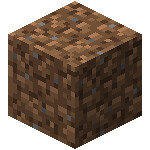In the image, there is a cube composed of numerous smaller interconnected cubes, forming a larger structure. The cube, with a distinctly scalloped edge, displays three of its faces. Each smaller cube varies in color, showcasing a spectrum from light blue and tan to different shades of brown, encompassing golden brown, bronze, and darker brown tones. Some pieces even have a nearly black or gray hue, adding to a complex, beautiful pattern reminiscent of granite, similar to what one might see on a kitchen countertop. The entire cube appears set against a clean, white background, lacking any other contextual elements to provide a sense of scale. The intricate combination of colors and shapes almost suggests a digitally rendered assembly applied to each face of the cube.